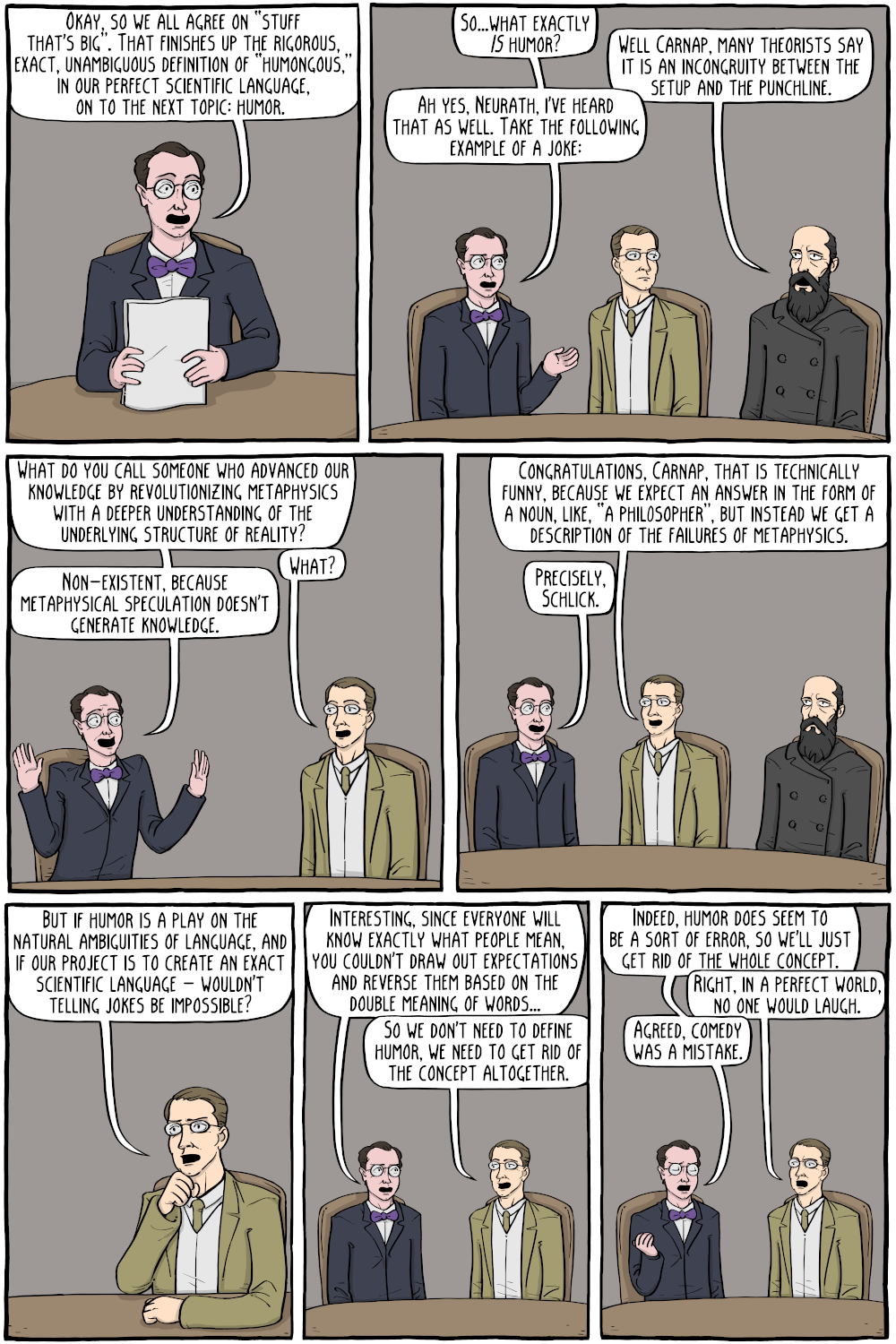In this seven-panel comic strip, the narrative begins with a bespectacled gentleman in a dark grey blazer, white shirt, and purple bow tie, holding some papers and seated at a table. He exclaims, "Okay, so we all agree on stuff that's big that finishes up the rigorous, exact, unambiguous definition of 'hormongous' in our perfect scientific language. Now, onto the next topic: humor." The scene then shifts to include two more men seated beside him—one in a green jacket with a vest and tie, also wearing glasses, and another in a dark grey, double-breasted blazer with a full beard and a bald head.

The gentleman in the purple bow tie initiates the discussion: "So what exactly is humor?" The bearded man responds, suggesting that humor is an incongruity between the setup and the punchline. This sparks a philosophical debate, with the purple-bow-tie man exemplifying a joke about the non-existence of metaphysical knowledge. The green-jacketed man congratulates him, analyzing the joke's play on language expectations.

As the panels advance, the man in the green jacket ponders whether humor, as a play on ambiguities in language, would be possible in their pursuit of a precise scientific language. The conversation concludes with the purple bow-tie gentleman asserting that in a perfect world, where everyone understands exactly what is meant, humor would be rendered unnecessary and thus obsolete. They agree that humor, and consequently comedy, was a mistake, culminating in their decision to eliminate the concept altogether.